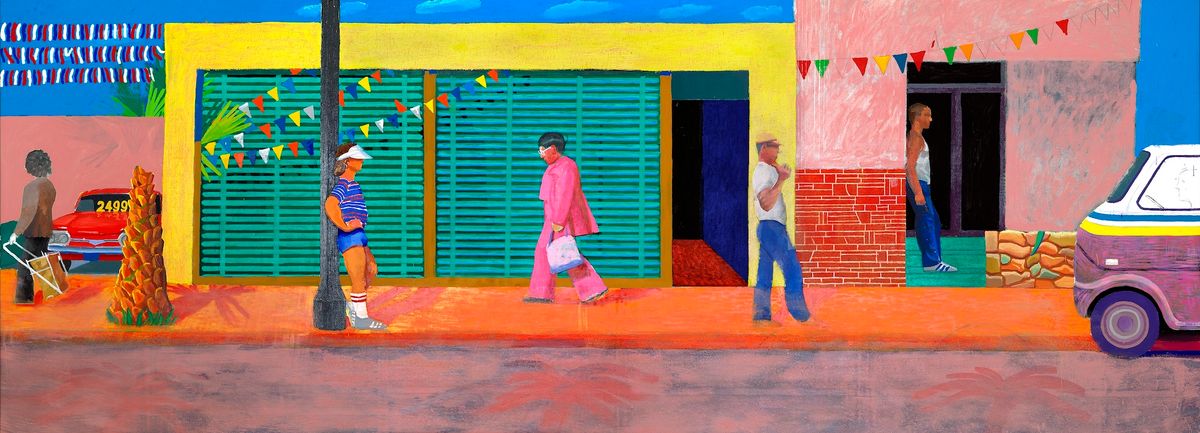The vibrant painting portrays a bustling city sidewalk bathed in bright tropical colors. The scene features an orange sidewalk lined with colorful buildings, including a prominent yellow building in the center with teal green double garage doors and strings of multicolored flags adorned diagonally across them. To the left of the yellow building, a pinkish structure has a unique combination of red brick and stone details at its base. 

Several people populate the sidewalk: a man leaning against a light post, dressed in blue striped shirt, blue shorts, gray shoes, white socks with red stripes, and a white visor; a woman in a pink outfit with short dark hair and white sunglasses, carrying a purse; another figure, pulling a grocery cart, clothed in a brown long-sleeved top and pants; and another man wearing blue jeans, a white tank top, and white shoes, standing within a turquoise-floored open doorway. Additionally, a man in blue jeans, white t-shirt, and a yellow cap strolls along the sidewalk.

Foregrounding the street scene, a purple van is parked to the right, adorned with yellow, blue, and white stripes, while farther left, a red car priced at $24.99 is discernible behind the stump of a palm tree. The clear blue sky overhead enhances the lively atmosphere, complemented by flying tassels and the colorful pennants fluttering in the breeze, evoking a warm, tropical ambiance reminiscent of places like Cuba.